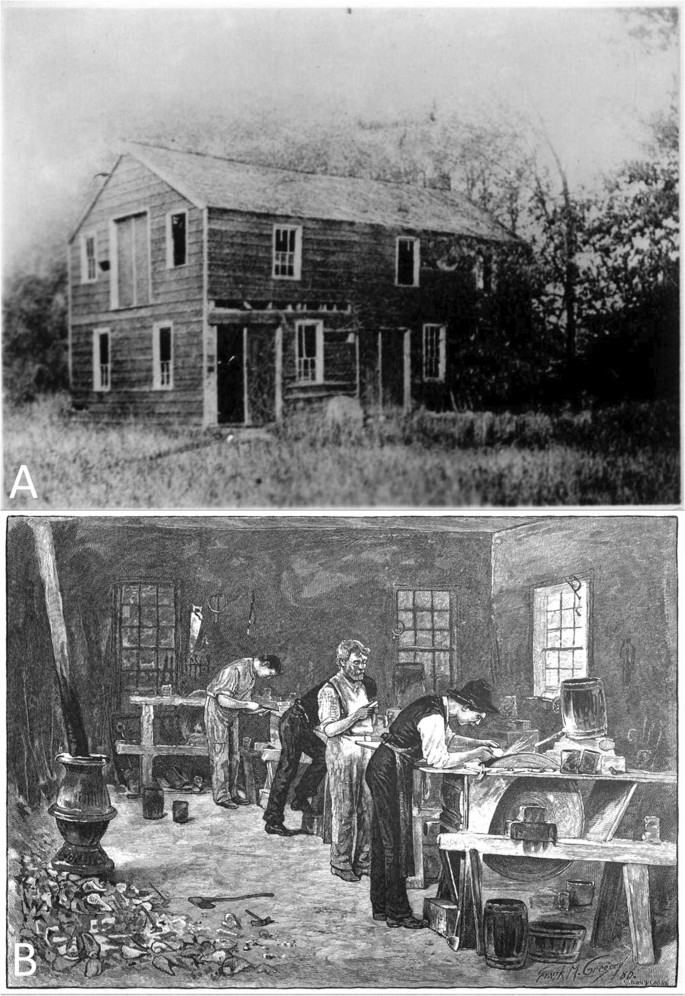The image has two labeled black-and-white components, labeled A and B. The top image, labeled A, is a photograph of a rustic, two-story wooden house, which appears to be from the 1700s or 1800s. It has nine visible windows and a door on the side facing the camera. The house stands alone in a grassy field, surrounded by trees, and exudes an aura of abandonment and wear.

The bottom image, labeled B, depicts the interior of a workshop, bustling with activity. Four men are shown standing and working at tables, most likely engaged in woodworking or metalworking. One man in particular is using a grinding wheel, with visible sparks indicating active sharpening or sanding. The workshop is cluttered with tools and debris, including axes on the floor, various tools on the walls, and a large urn to the left. The room is lit by three windows, through which daylight streams, casting light on the industrious scene within.